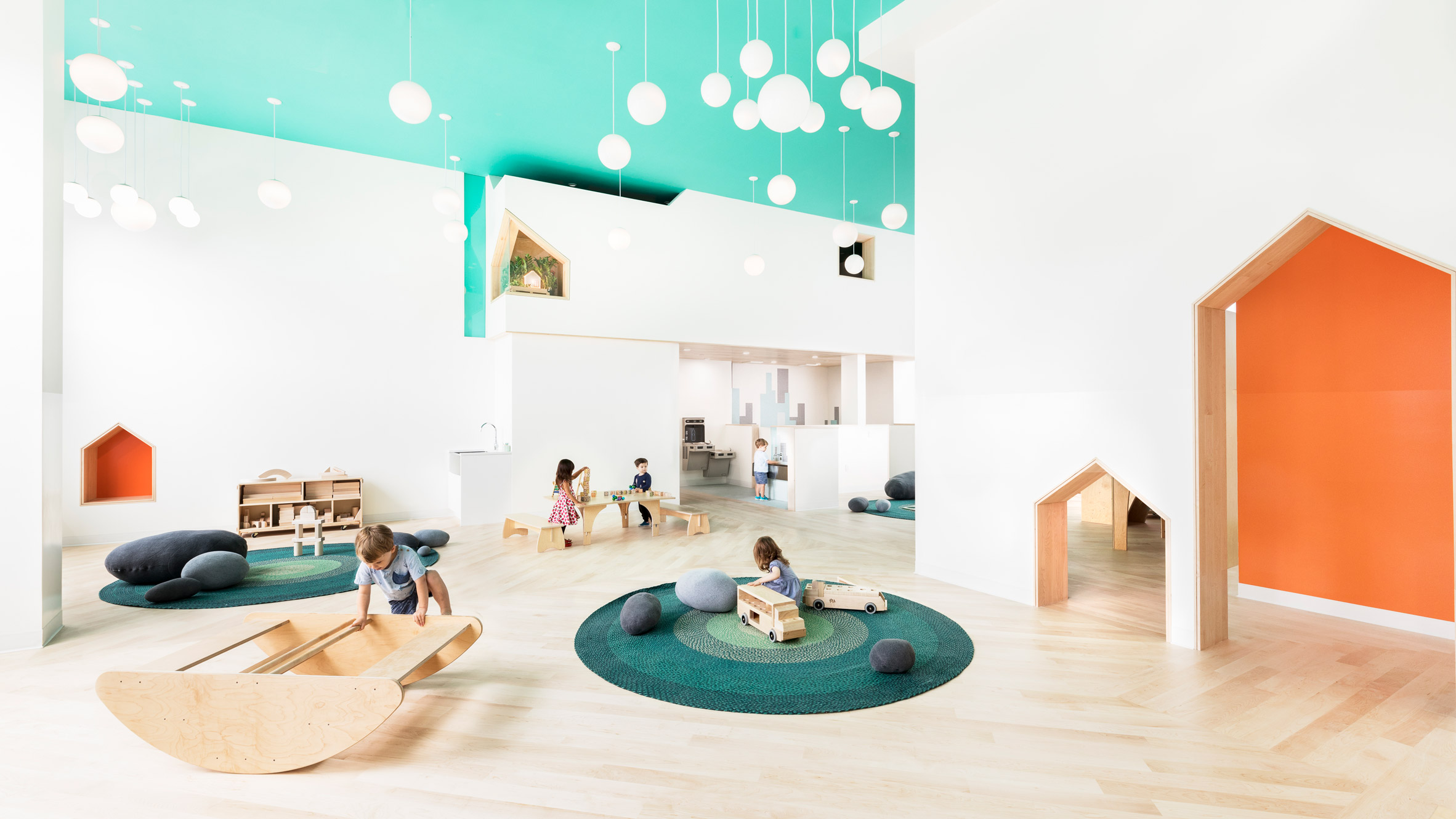The photograph showcases a modern children's play area with 20-foot ceilings and a light blue to green gradient walls, accented with an orange section. The spacious area features a light hardwood floor and numerous play stations. Several children are seen engaging in various activities. Some are playing on circular green rugs with pebble-shaped pillows, while others are near a seesaw-like wooden table with half-moon shapes. White circular light fixtures and large white architectural fixtures hang from the ceiling, adding a bright and airy feel. In one section, a child is playing with a wooden truck, and another is on a blue-green circular carpet with pillows, playing with a toy bus. Near a bookshelf with a reading nook, a boy plays with a wooden rocking boat, and a boy and girl appear to be playing "restaurant" at a small table. Arched house-shaped wall cutouts add playful architectural interest to the vibrant and engaging environment.